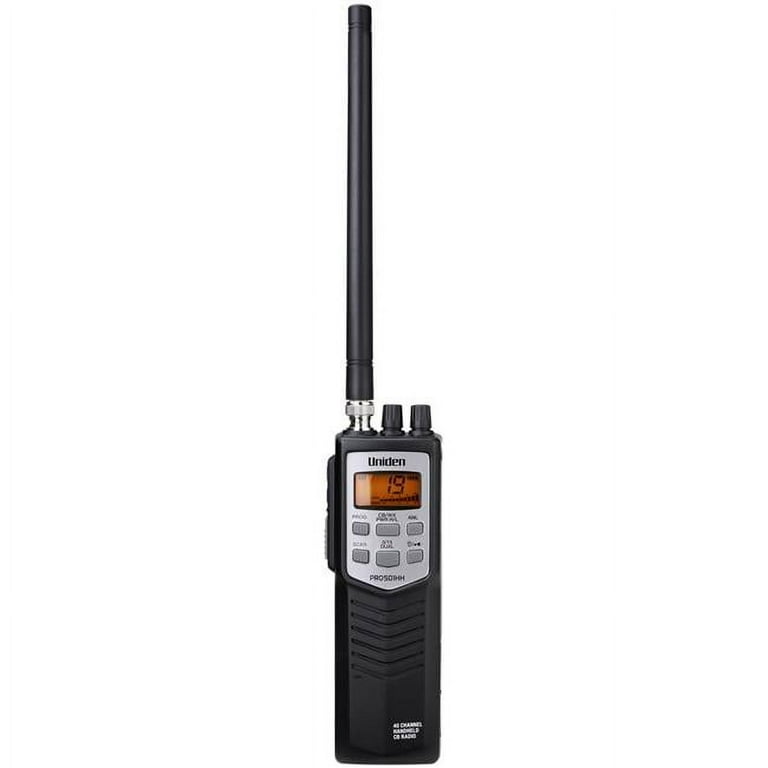The image depicts a Uniden brand walkie-talkie, identifiable by its logo displayed above the electronic screen. The device, primarily black, features a sturdy and elongated black antenna attached on the left side, approximately 16 inches tall. The walkie-talkie is about 10 inches in height and includes a pair of control dials positioned on the top of the unit, located in the middle and right side. The digital display, which shows the number "19" with an intensity bar beneath it, has an orange background. Below the display, there are six buttons arranged in two rows of three. Additionally, there are push-to-talk buttons on both the left and right sides of the device and a black base, likely designed for grip. Some text at the bottom of the walkie-talkie is partially legible, suggesting it might be labeled with terms like "radio" or "one channel."